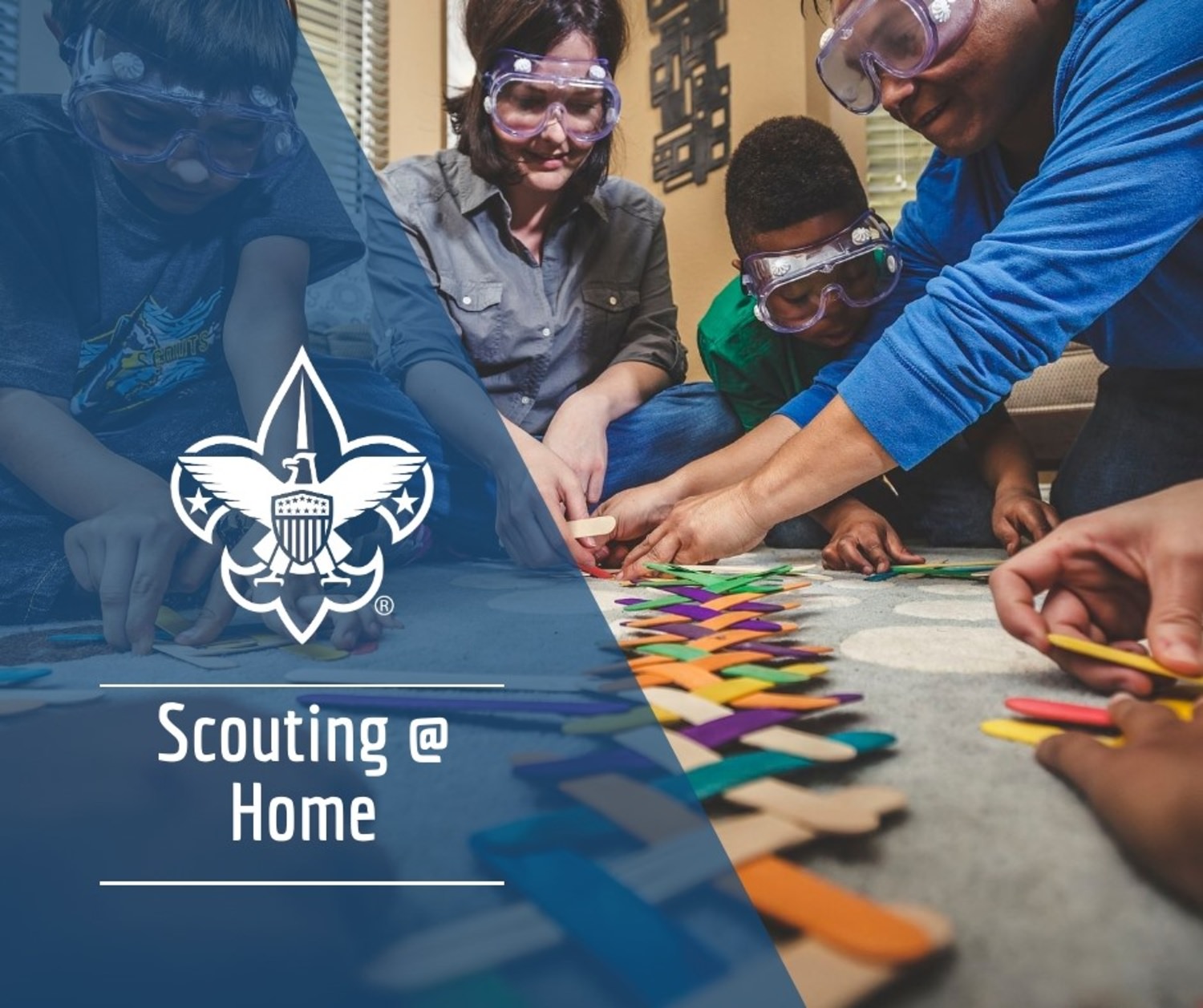The horizontal rectangular advertisement for a scouting organization is divided diagonally from the top left corner to about the middle, creating a semi-transparent blue triangle overlay on the left side. Within this blue section, there is a logo featuring an eagle with plant-like details and stars beneath its wings, accompanied by the white text "Scouting at Home" framed by lines above and below the text.

On the right side of the image, a colorful and detailed photograph captures a family engaged in a craft project. The scene includes a woman, a man, a child, and the hands of another person who is out of frame. All visible individuals are wearing protective goggles. The project they are working on appears to involve thin strips of wood, characterized by a vibrant color palette that includes tan, white, black, brown, bright blue, purple, orange, yellow, green, and gray. The overall layout suggests a structured presentation designed to promote at-home scouting activities.